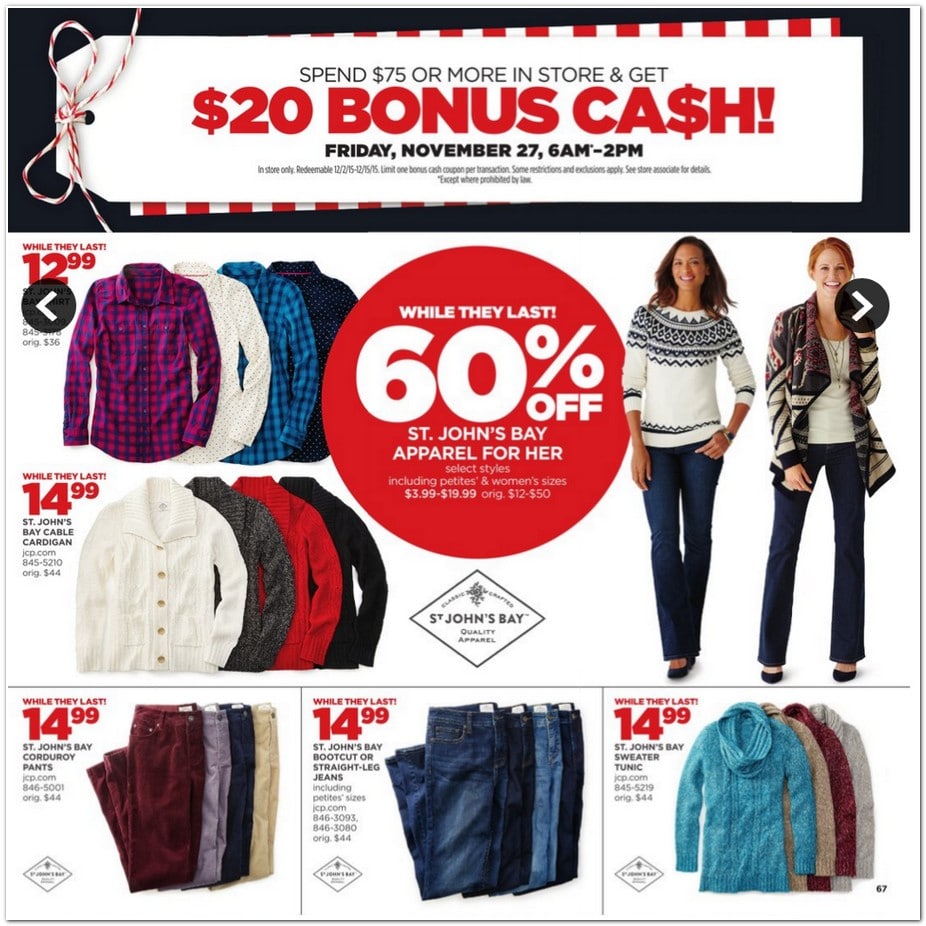This promotional flyer for a sale prominently features a black header showcasing a large white price tag adorned with a red and white bow on the left side. The text on the tag reads, "Spend $75 or more in-store and get $20 bonus in cash," with the "$20 bonus in cash" written in large, bold, red all-capital letters, with the word "cash" indicated by a dollar sign.

Directly below this, the timing details are specified: "Friday, November 27th, 6 a.m. to 2 p.m." Beneath these details, in fine print, it states: "In-store only. Redeemable 12/2/15 through 12/15/15. Limited to one bonus cash coupon per transaction. Some restrictions and exclusions apply. See store associate for details. Except where prohibited by law."

The central focal point of the flyer is a prominent red circle with white text announcing a "60% off" sale on St. John's Bay apparel for women. This sale includes various styles, including petite and women's sizes, with prices ranging from $3.99 to $19.99, originally priced from $12 to $50. The "60% off" text is the most eye-catching element.

To the left of this main promotion are images of several women's long-sleeve shirts priced at $12.99 and $14.99. An emblem for "St. John's Bay Quality Apparel" is also centrally displayed.